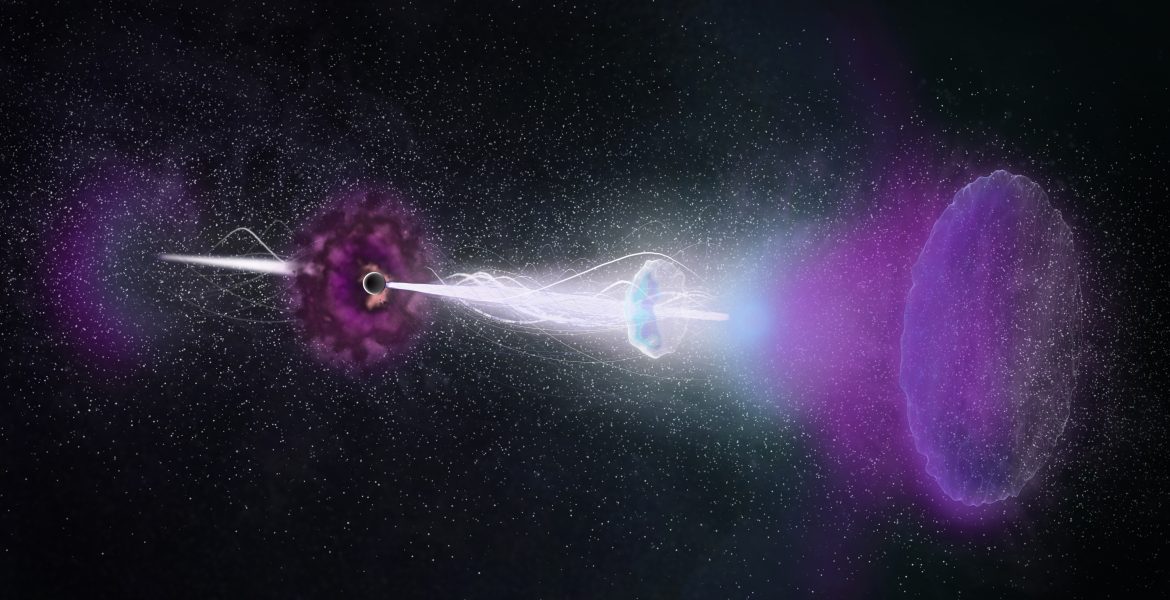The image appears to be an artist's rendering of a dramatic event in space, set against a dark black backdrop filled with countless white stars. At the core of the image is a dynamic scene dominated by a vivid contrast of colors and forms. Situated slightly to the left of center, a purplish, gaseous-like diffusion emanates from a black hole, suggesting the intense gravitational forces at play. Piercing through this purple mass is a brilliant, white beam of light that seems to be emerging post-explosion, resembling a trumpet-like projection. White wavy lines of energy streak through this hole, adding to the sense of chaotic power and motion. The artistic style leans heavily towards science fiction, evoking imagery of phenomena such as wormholes or hyperdrive travel, with the tendrils and lens-like shapes contributing to the surreal, otherworldly atmosphere.